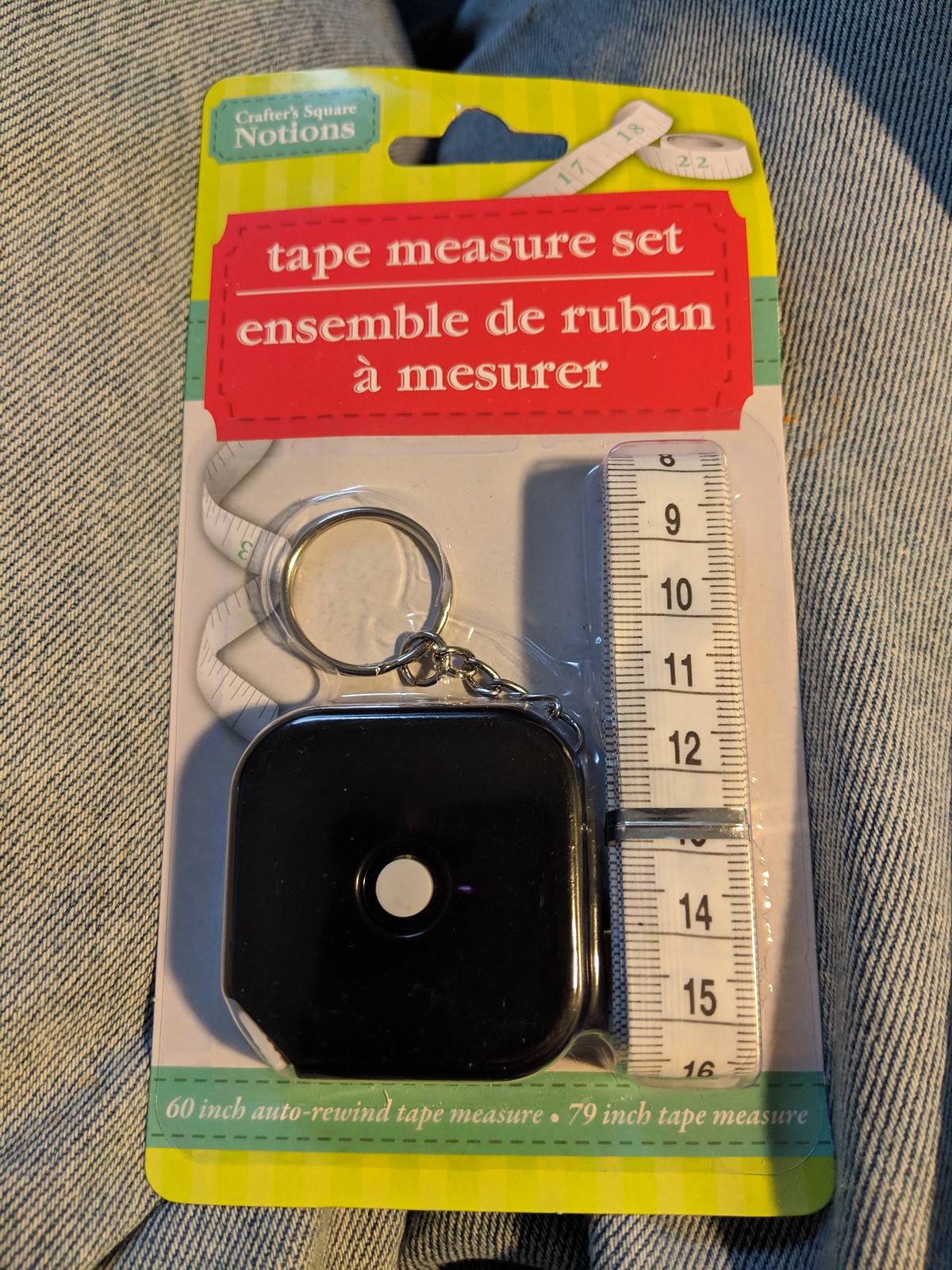The image depicts the packaging of a tape measure set, prominently centered in the photograph. The package, made of cardboard and covered in plastic, showcases a tape measure and a soft-backed measuring tape. The cardboard label is vibrant and eye-catching, predominantly yellow with green and white accents. At the top, a small green square with an illegible brand name is noticeable. Below this, a large red rectangle with white text indicates the product name in both English and French, "Tape Measure Set" and "Ensemble de Ruban à Mesurer," respectively. The red section is bordered by a decorative tape measure graphic stretching to the black square tape measure.

On the upper left, a green ticket stub-like label reads "Notions," while on the bottom, the detailed product specifications display "60-inch auto rewind tape measure" and "79-inch tape measure." The black square housing, located in the bottom left, contains the tape measure and is equipped with a silver steel keychain. The white tape measure, visible to the right of the square housing, has numerals ranging from eight to sixteen, with precise measurement lines. The package sits atop a piece of pinstriped fabric, adding to the aesthetic presentation.